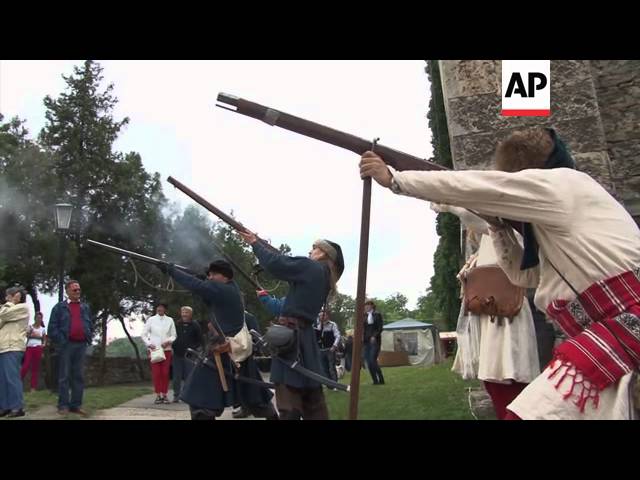The image is a color photograph in landscape orientation, depicting a historical reenactment scene set in a grassy field. The photograph captures several individuals dressed in period costumes reminiscent of the 1600s, portraying hunters, trappers, settlers, and native figures. The rightmost figure, closest to the viewer, is clad in a long-sleeved white tunic with a red striped blanket tied around their waist, their face obscured by their raised left arm as they aim and fire a long rifle resting on a wooden support. Adjacent to them, another figure in a white dress with a dark brown saddlebag over their shoulder similarly aims a musket skyward.

In the center of the image, a group of men dressed in dark clothing, including long blue coats, hold and fire rifles in a curved line pointing towards the top left of the image. Notably, two individuals on the far right wear native attire, consisting of long white shirts and traditional accessories such as a leather pouch and a Davy Crockett-style hat.

In the left section of the image, two spectators can be seen: a man in a dark jacket with a red undershirt and pants, and a woman with her back turned, wearing a white jacket and blue pants. Thin black bars run across the top and bottom of the image, which features the AP logo (a white rectangle with a red line at the bottom and black "AP" text) in the upper right corner, suggesting it is part of a documentary or report.

Background elements include pop-up tent structures that evoke an outdoor Renaissance Faire or a 1600s battle reenactment, enhancing the scene's historical ambience. The overall visual style is photographic representational realism.